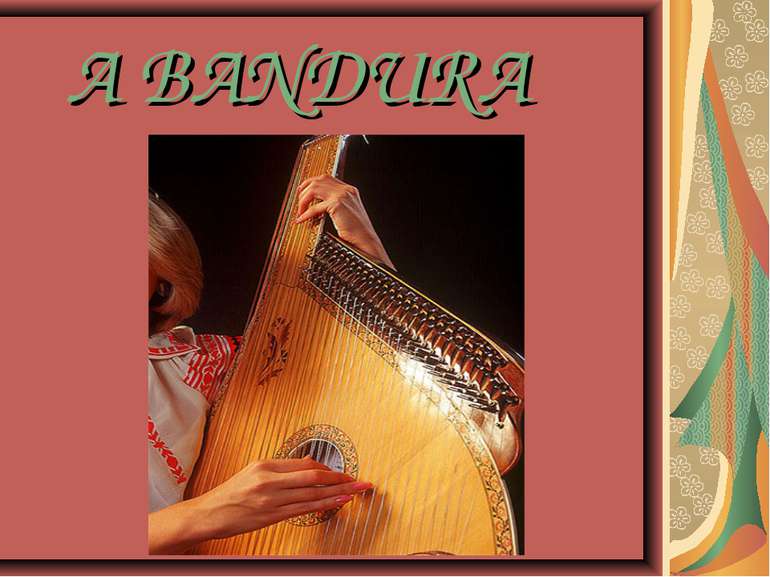The digitally enhanced landscape-oriented photograph features a woman playing a Mexican-style string instrument that resembles a guitar but is larger, held upright, and more intricate. Her face is not visible as it's cut off on the left side of the image, but you can see her blonde, short hair and feminine hands with pink nail polish. She wears a red and white Mexican-style dress. The background of the image is a pinkish-orange hue, and the border around the photograph is thick and pink. At the top, in teal script font, the text reads "ABANDURA," suggesting this could be an album cover. Along the right side of the photograph, there is a vertical strip with a floral design in various colors including sage, orange, and light yellow, adding to the overall decorative aesthetic.